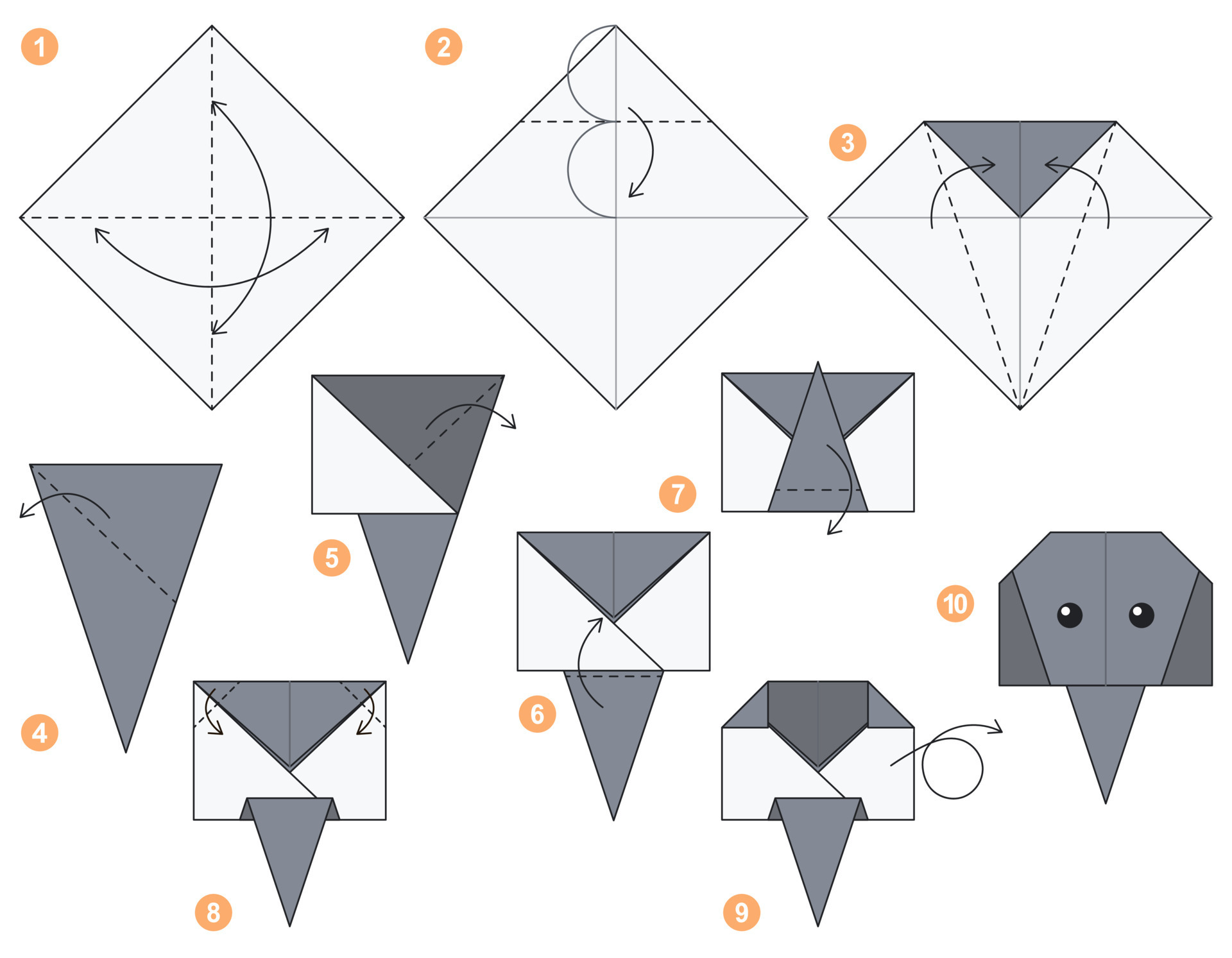This image is a detailed diagram depicting instructions on creating an origami elephant head. The step-by-step guide consists of ten numbered illustrations, each marked by a small tangerine-colored circle containing white numerals. The diagram uses a white background with black solid and dotted lines to indicate fold lines and arrows to show the direction of the folds.

The process begins with a flat piece of paper, transitioning through a series of precise folds. The illustrations show gray shading on folded sections to contrast with the remaining white areas, helping to visualize the progress. Initially, the paper is folded into quarters, then into a diamond and triangular shapes, progressively shrinking in size.

Throughout steps 1 to 10, the distinctive features of the elephant gradually emerge, including its trunk and ears. The final step reveals a fully formed elephant head, complete with eyes. This thoughtfully illustrated guide provides a clear, visual narrative for transforming a simple piece of paper into a charming origami elephant.